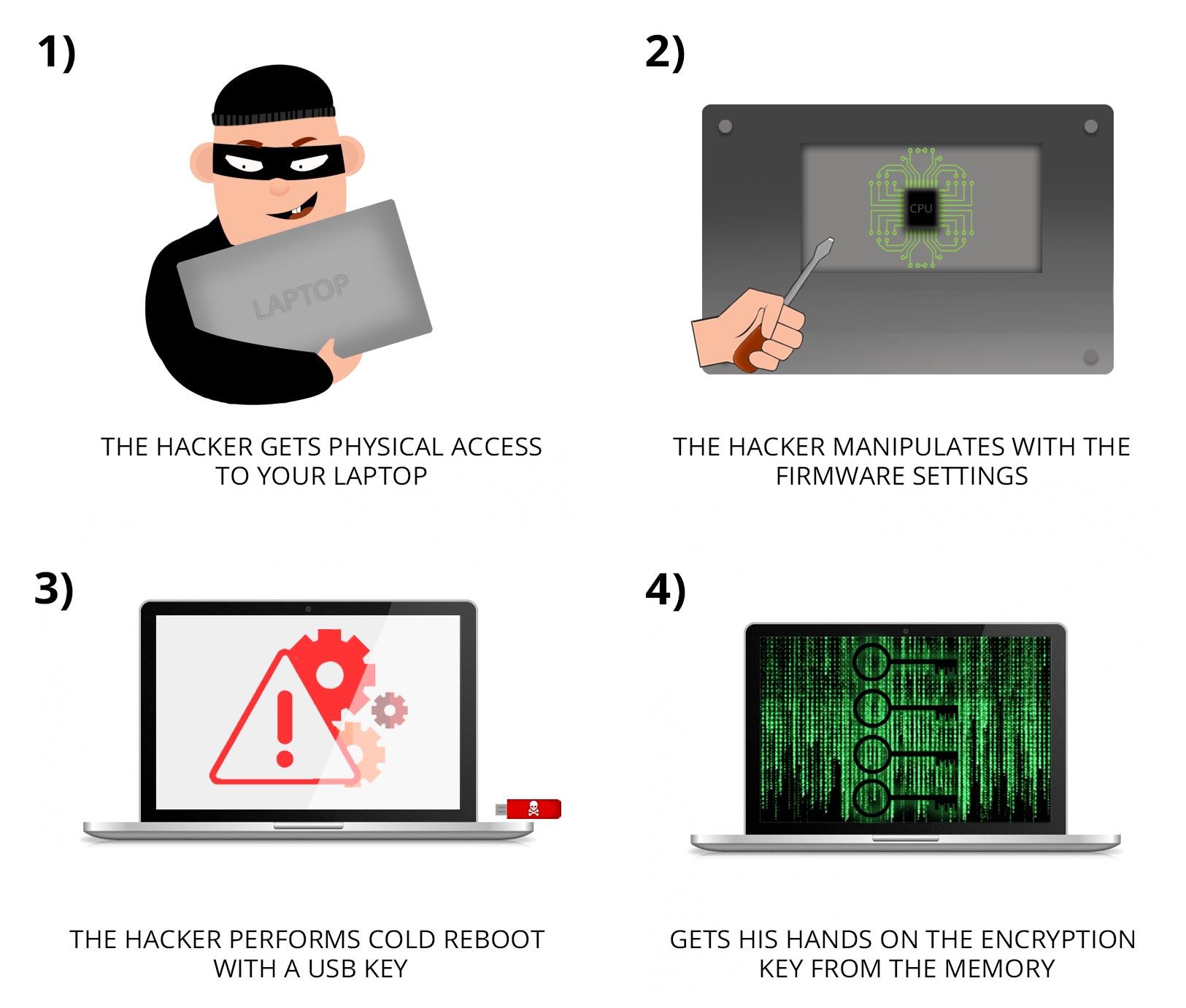This infographic illustrates the step-by-step process of how hackers infiltrate a laptop using a cartoon-like square grid format with a light background. The top-left section is marked "1" and depicts a stereotypical comical criminal with light skin, wearing a black beanie, black eye mask, black sweater, and holding a grey laptop labeled "Laptop." The accompanying text states, "The hacker gets physical access to your laptop." In the top-right section, labeled "2," a hand with a wooden-handled screwdriver is shown near a metal-based CPU with the text, "The hacker manipulates firmware settings." In the bottom-left section, marked "3," a laptop screen displays a red triangle, exclamation point, gear symbol, and USB key adorned with a skull and crossbones, indicating, "The hacker performs cold reboot with a USB key." The bottom-right section, labeled "4," shows a laptop with famous "Matrix-style" streaming green letters and numbers, conveying that the hacker, "gets his hands on the encryption key from the memory."